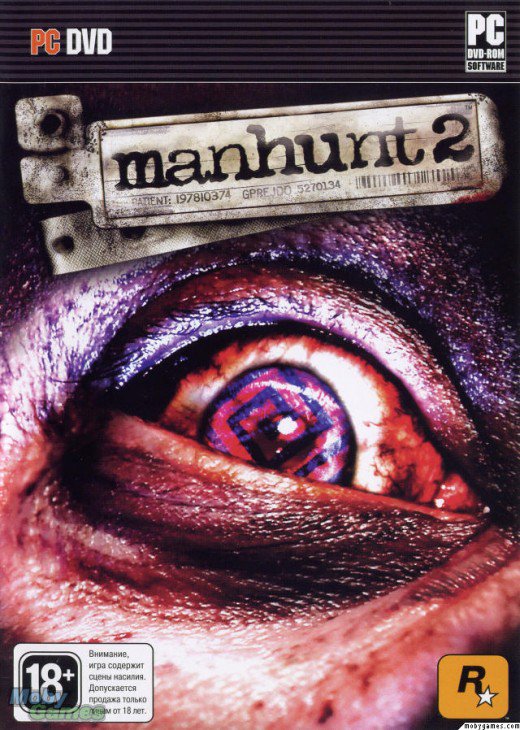The image is the cover of a PC DVD-ROM software for the video game "Manhunt 2". Dominating the cover is a highly detailed, zoomed-in picture focusing on the right eyeball of an older person. The eye, marked by fine lines and wrinkles, indicates wear and tear from age and stress. The eyeball itself is fascinating and somewhat disturbing; it is predominantly red, with only a small portion of white around the iris and pupil. Intriguingly, there is a spiral of red and blue running through the center, giving the eye a stressed and terrified expression. The face surrounding the eye is generally red in color. At the top, the title "Manhunt 2" is prominently displayed along with the text "patient 197810374" and a barcode. Additional details include the "18+" age rating at the bottom, the PC DVD-ROM software label at the top right, and the Rockstar Games logo on the right side. This highly stylized cover uses a mix of colors including black, gray, white, red, tan, purple, blue, and green, all contributing to its unsettling and intense appearance.